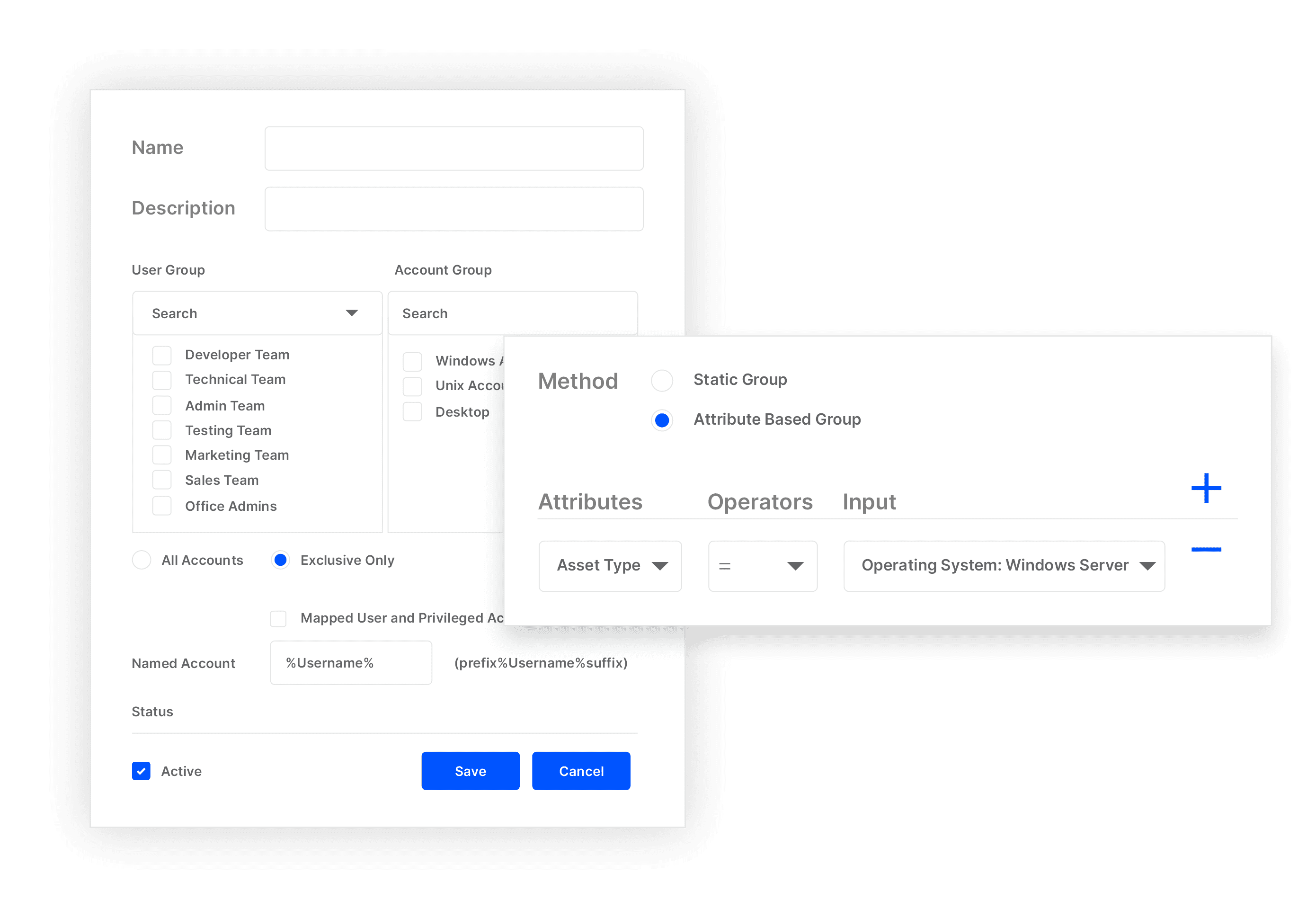The image features two juxtaposed sections, intricately detailed with various fields and controls. On the left side, the top showcases the word "Name" followed by an elongated rectangular input field stretching to the right. Below that, a similar configuration exists with the label "Description" above another extended rectangular field. Further down, the label "User Group" is followed by a smaller rectangular box with the word "Search" inside, accompanied by a rightward arrow pointing downwards. Beneath this, a vertical list in black text displays user group categories: "Developer Team," "Technical Team," "Admin Team," "Testing Team," "Marketing Team," "Sales Team," and "Office Admins."

Mirroring this structure on the right side, the section is headed by "Account Group," beneath which a small rectangle also labeled "Search" exists, followed by categories "Windows" and "Unix Desktop." There is an overlapping rectangular field that extends across the right side and contains all account options, flanked by indicators for "Exclusive Only" marked by a blue dot. Below this are fields for "Name Account," "Username," and "Username Suffix," followed by a status indicator. In the bottom left corner, a blue square with a white check mark denotes "Active," while the bottom right corner houses two blue buttons with white text: "Save" on the left and "Cancel" on the right. 

The overlapping tab at the top left includes the header "Method," with "Static Group" to its right. Below that, options for "Attribute Based Group" are marked with a blue dot. The left section reads "Attributes and Operators and Input," segmented by a blue plus sign above a blue dash. On the right side of this tab, the label "Operating System Windows Server" is visible, followed by "Asset Type" on the left with a dash and an upside-down triangle. 

The entire design features slight shadowing along the sides, adding depth to the layout.